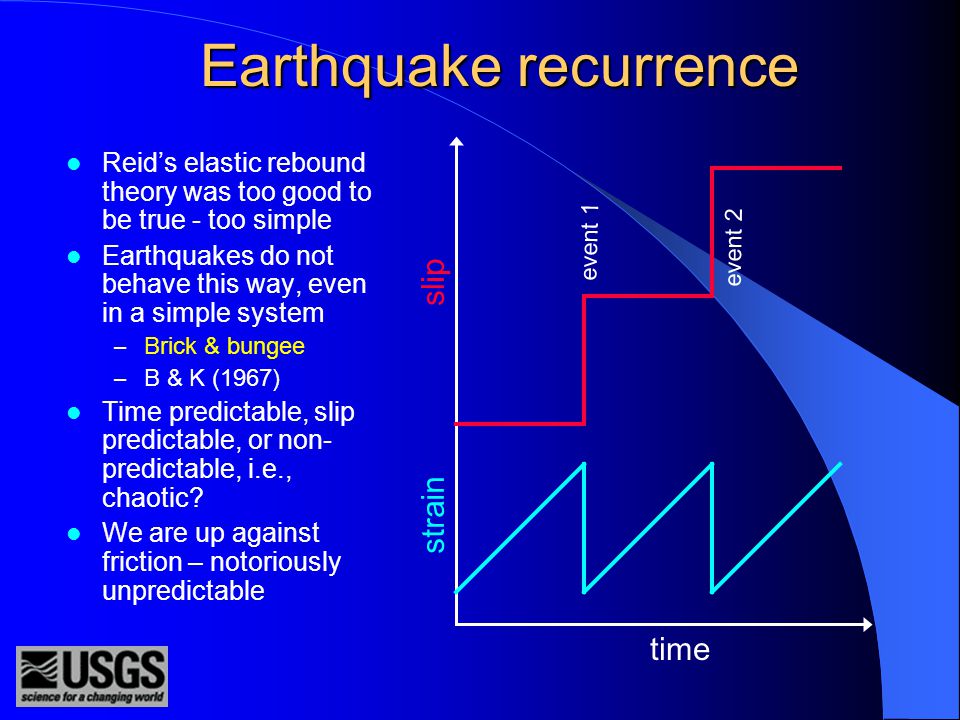The image is a detailed screenshot of an educational PowerPoint presentation on earthquake recurrence, featuring a blend of text and a graphic against a gradient blue background that darkens from left to right. At the top, in beige letters, it prominently displays the title "Earthquake Recurrence." On the left side, clearly outlined in white with light blue bullet points, are the key points: "Reed's elastic rebound theory was too good to be true, too simple. Earthquakes do not behave this way, even in a simple system. Birkin-Bungee, BNK 1967. Time predictable, slip predictable, or non-predictable, i.e., chaotic. We are up against friction, notoriously unpredictable." 

On the right side, there is an informative graph that includes an aqua-colored sawtooth line at the bottom, representing strain over time, and a red staircase-like line above it indicating different seismic events, labeled "event one" and "event two." The y-axis is marked with the term "strain" in light blue, while the x-axis at the bottom is labeled "time." The bottom left corner features the logo and tagline of the United States Geological Survey (USGS), stating "Science for a changing world." The overall design uses a combination of colors including blue, white, light blue, gray, black, red, and yellow, ensuring visual clarity and emphasis on key information.